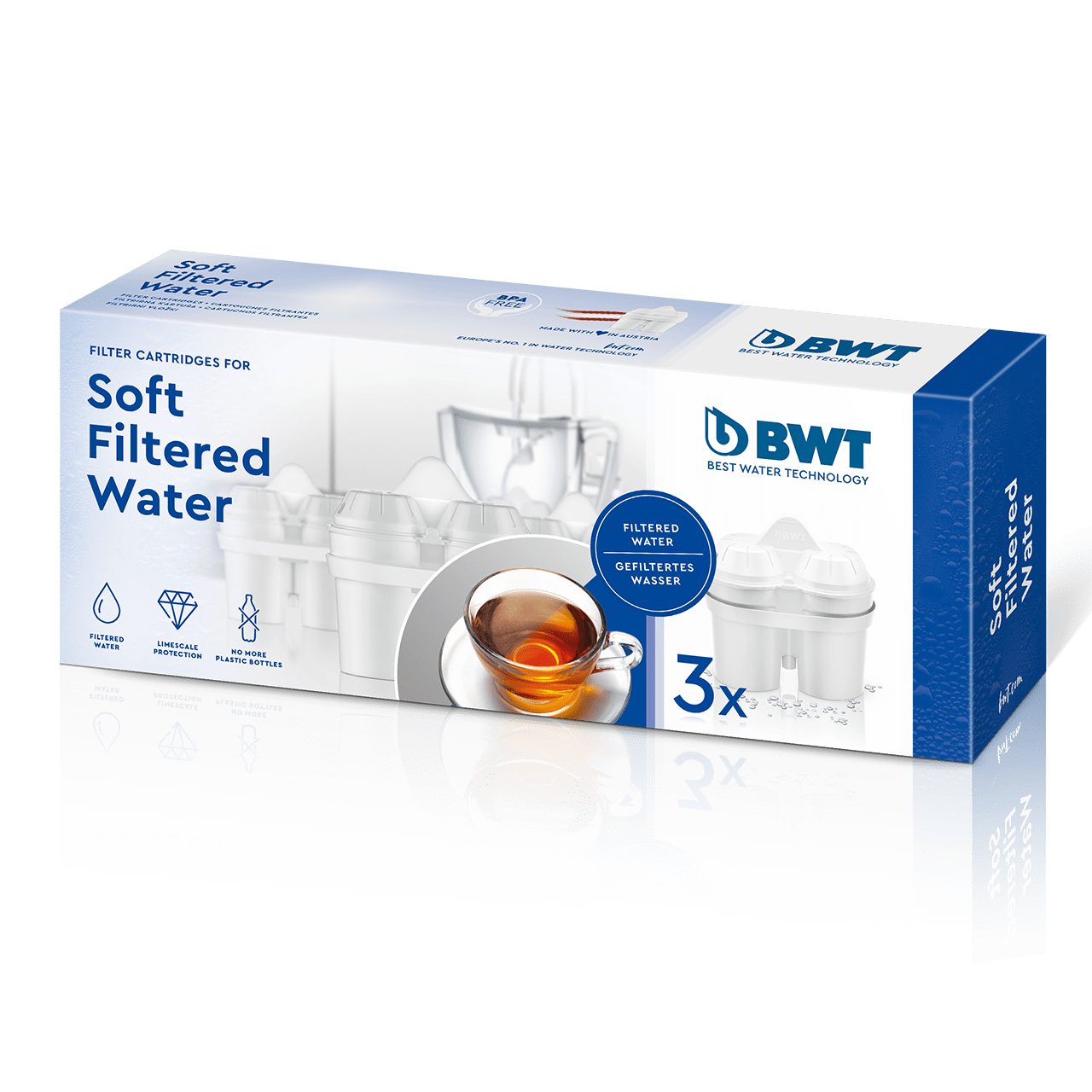The photograph depicts a horizontally-oriented box for soft filtered water products, centrally positioned against a shiny white background that reflects the box beneath it. The box appears new and sealed, suggesting that the filters inside are unused. The box is predominantly light white with bluish gray tones and incorporates various visual and textual elements to detail its contents and benefits. 

In the middle of the package, there's an image of three filter canisters, each with a clear top, alongside a clear glass teacup filled with amber-colored tea, resting on a saucer. Nearby, a blue circle contains multilingual text indicating "filtered water," "g-filter test," and "wasser," with a large "3X" next to it. 

The upper left section features the text "Soft Filtered Water" in bold blue lettering, preceded by "Filter Cartridges For" in smaller text. Below this title, three graphic symbols represent filter benefits: a water droplet labeled "Filtered Water," a diamond symbol signifying "Limescale Protection," and a crossed-out wine bottle indicating "No More Plastic Bottles." 

In the upper right corner, the brand name "BWT" is prominently displayed in capital blue letters, with the tagline "Best Water Technology" beneath it in smaller text. The design includes a solid blue vertical stripe on the right side of the box, with sideways white text reiterating "Soft Filtered Water."

The style of the image aligns with photographic realism, often seen in product photography for lifestyle or home product networks.